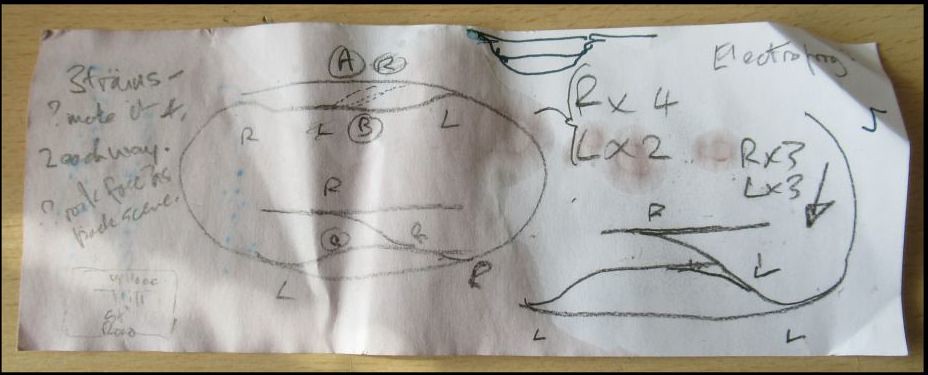A large sheet of white paper lies on a light wooden background, partially water-damaged on the left side. The content is handwritten in black ink, though some of the writing is difficult to discern.

On the left side, where the damage is more severe, there is a visible number "3" followed by what appears to be "FRAUS-" and several lines of text beneath it. Lower down, there is a square with additional writing inside. A large circle containing assorted letters encircled and connected with lines occupies the middle of the page. At the top, an interesting shape resembling a teacup is drawn.

The right side of the paper, which is less affected by water, includes notations like "RX-4," "LX-2," "RX-3," and "LX-3," along with an arrow pointing downward and assorted lines. In the upper right corner, the paper is folded slightly, and the word "ELECTRO" is partially visible, though the rest is not legible due to the fold.